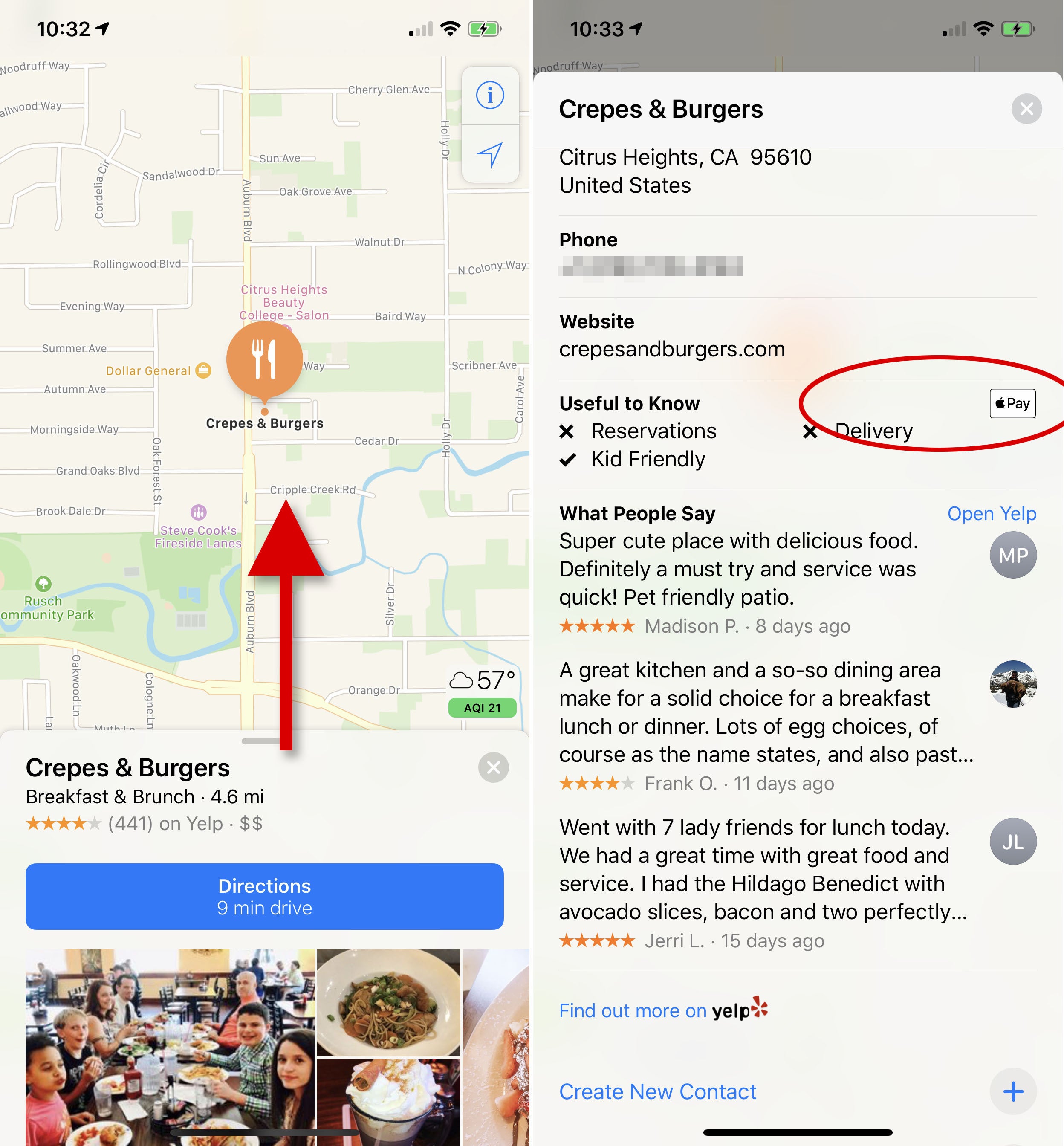A photo captures a Yelp page on a smartphone displaying details for the restaurant "Crepes and Burgers," a breakfast and brunch spot rated 4 stars from 441 reviews. The listing indicates the establishment is moderately priced, denoted by two dollar signs ($$). The screen shows a "Directions" button, noting a nine-minute drive from the user's current location. A map beneath the directions includes a red arrow pointing to the restaurant's location in Citrus Heights, California. To the right of the map, a red oval highlights the availability of "Delivery" and compatibility with "Apple Pay." The detailed information includes the restaurant's website, crepesandburgers.com, while the phone number is blurred for privacy. The page mentions that while the restaurant does not accept reservations, it is kid-friendly. Three user reviews are also partially visible at the bottom of the screen.